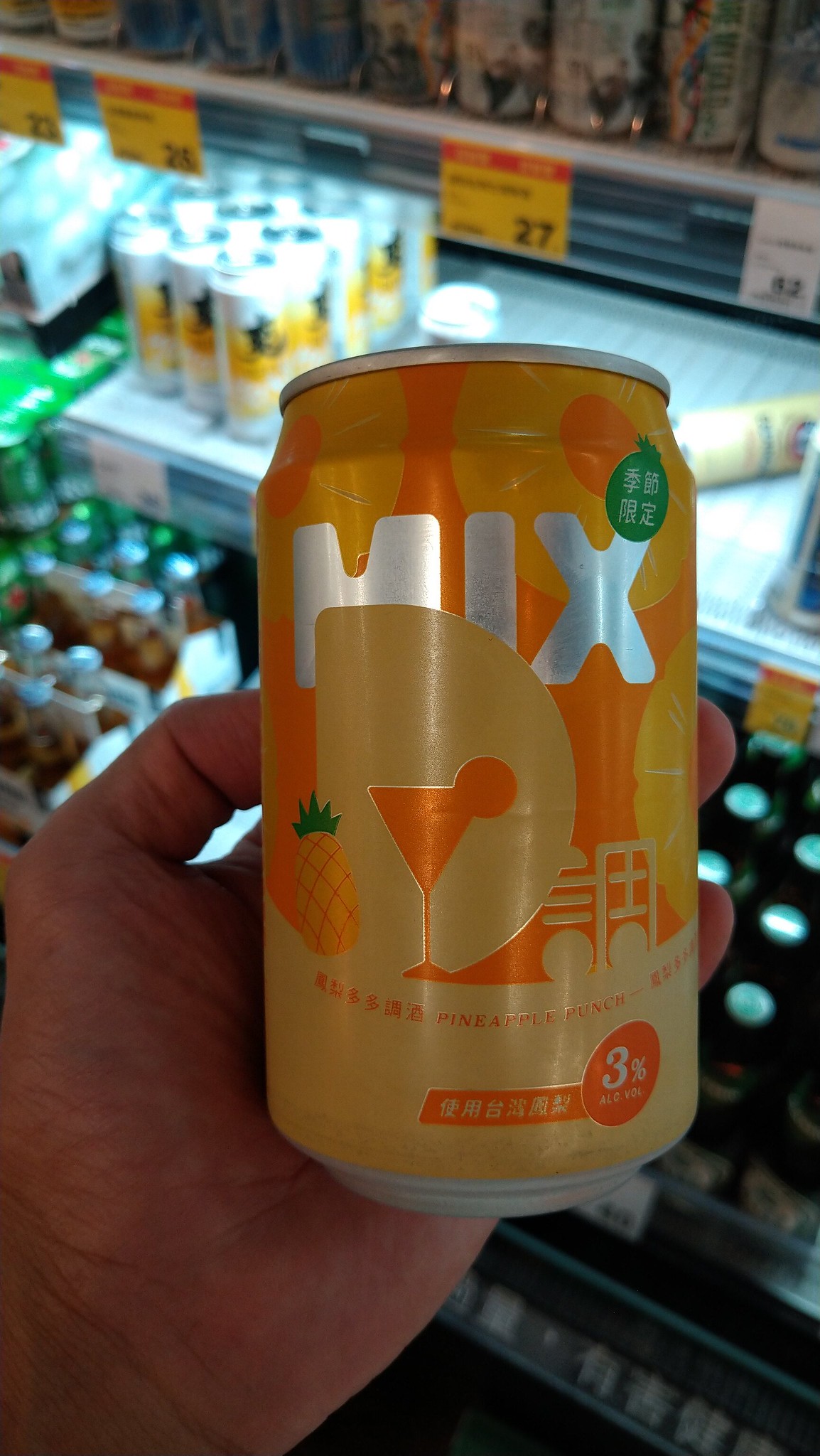In this vivid image, a person’s hand is prominently positioned in the bottom left corner, securely holding a cylindrical can. The can's design is striking, with its circular top and bottom clearly defined. The can's side is primarily adorned with vibrant hues of orange and yellow, creating a bold visual impact. On the top right of the can, a cluster of white foreign characters stand out against a lush green background, adding an exotic touch to the design. Beneath this, the word "MIX" is displayed in a sleek silver font, easily catching the eye. Further below, to the left, a detailed artwork of a pineapple adds a playful yet tropical element to the can's aesthetic. The bottom portion of the can transitions into a gradient of warm orange and red tones, completing the colorful and dynamic design.